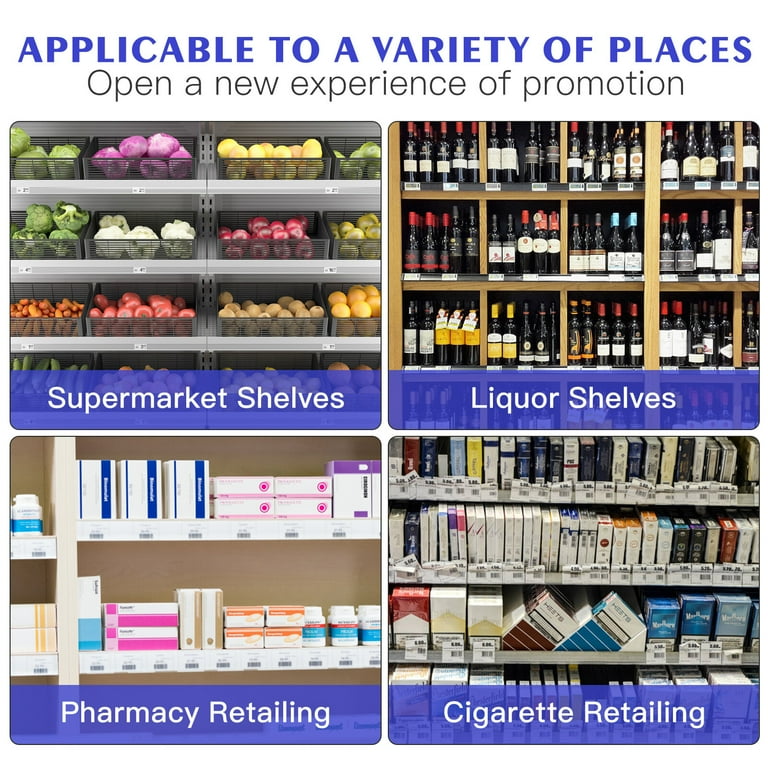The poster, titled "Applicable to a Variety of Places: Open a New Experience of Promotion," showcases four distinct retail shelving layouts, each designed for different types of stores. The top left quadrant, labeled "Supermarket Shelves," displays assorted fruits and vegetables meticulously arranged on supermarket shelves. The top right quadrant, labeled "Liquor Shelves," features an array of wine bottles neatly stacked. In the bottom left, the "Pharmacy Retailing" section shows shelves lined with various medicine boxes and bottles. Finally, the bottom right section, "Cigarette Retailing," depicts shelves stocked with numerous cigarette cartons, exemplifying an organized smoke shop. Each quadrant provides a visual representation and label of how products can be attractively and efficiently displayed to enhance promotional efforts in diverse retail settings.